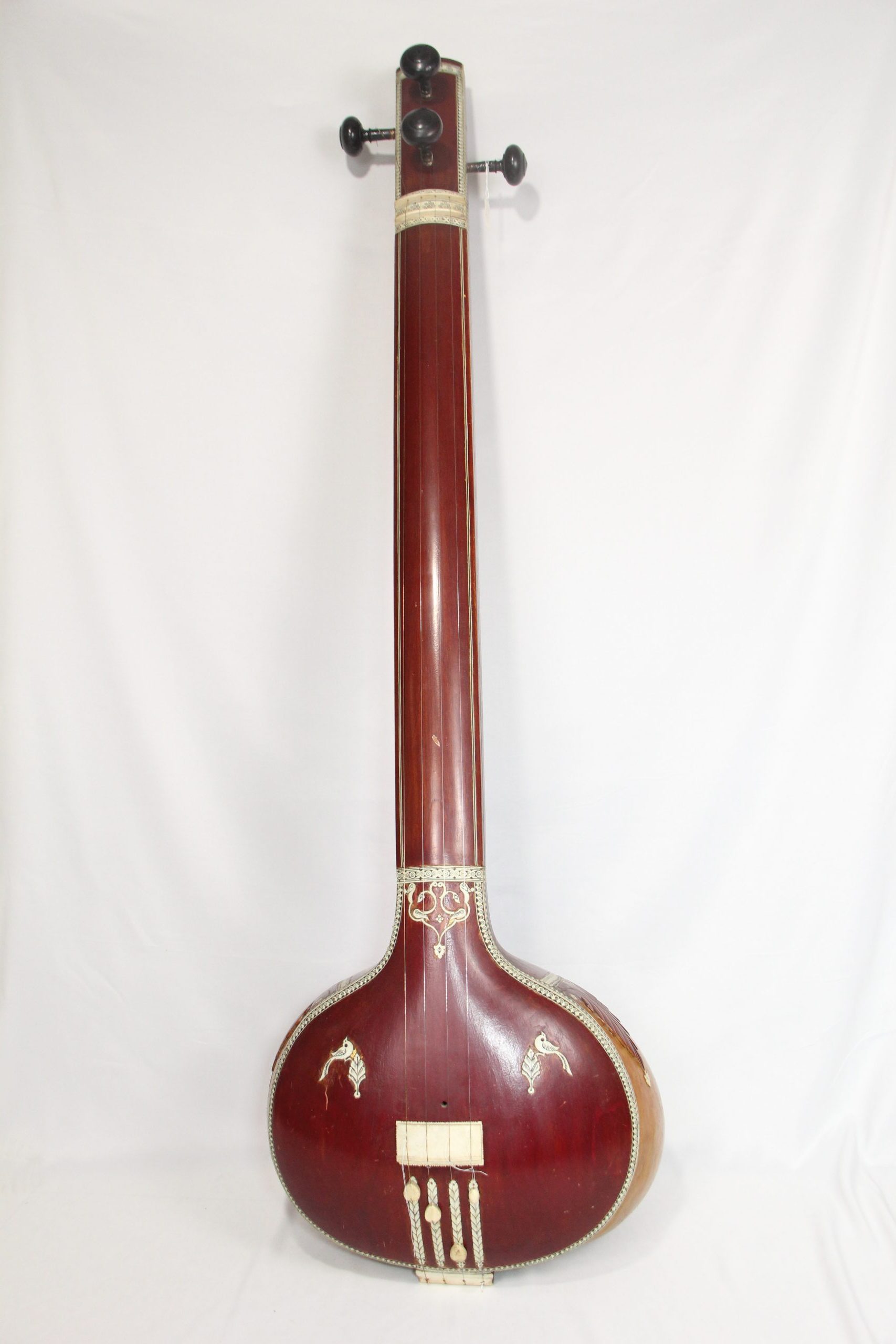This image showcases a beautifully crafted musical instrument against a white backdrop, spanning the entire height of the vertical frame. The instrument features a rich, mahogany reddish-brown body resembling a halved melon or a bulbous thermometer at the bottom. It has a beige rim and a thin white line running along its edges and sides. The back of the instrument shows a detailed tan scroll decoration. The long neck extends seamlessly from the bulbous bottom to the top, where four black pegs are prominently visible—two positioned vertically in the center and one on each side. The instrument, suspected to be of Asian origin, might resemble a sitar or a similar stringed instrument, with its four visible strings and ornate craftsmanship.